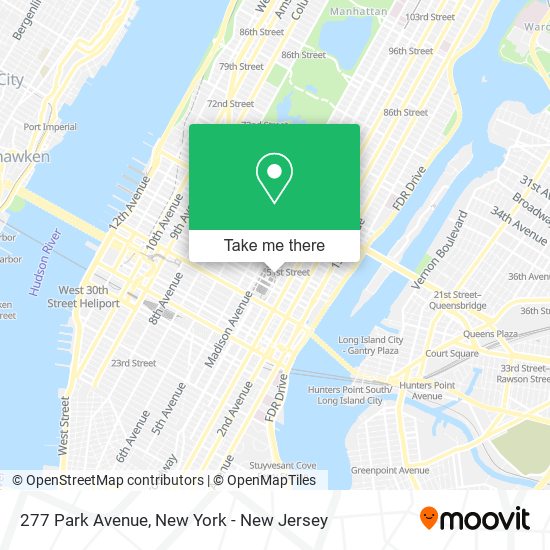This image features a detailed map screen prominently displayed. In the bottom right corner, the logo "MOOVIT" (spelled M-O-O-V-I-T) is visible with an orange balloon icon to its left. Adjacent to this logo is the address "277 Park Avenue, New York-New Jersey." Slightly above, credits are given to "OpenStreetMap contributors" and "OpenMap tiles."

The map displays three distinct sections of the city, separated by bodies of water, with the land areas depicted in gray and the water in blue. From left to right, the pattern alternates between gray (land) and blue (water), ending with a gray section on the right. Various locations and roads are identified with black text. The viewpoint is a downward perspective, as if looking from above. Green spaces are scattered at the top of the map, particularly around the city of Manhattan.

In the center of the image, there's a prominent visual with a tall building, estimated to be 30 to 40 stories high, against a light blue sky. This visual is paired with the caption "Take Me There" written in blue text and is specifically pointing to 15th East Street, which is centrally located on the map.